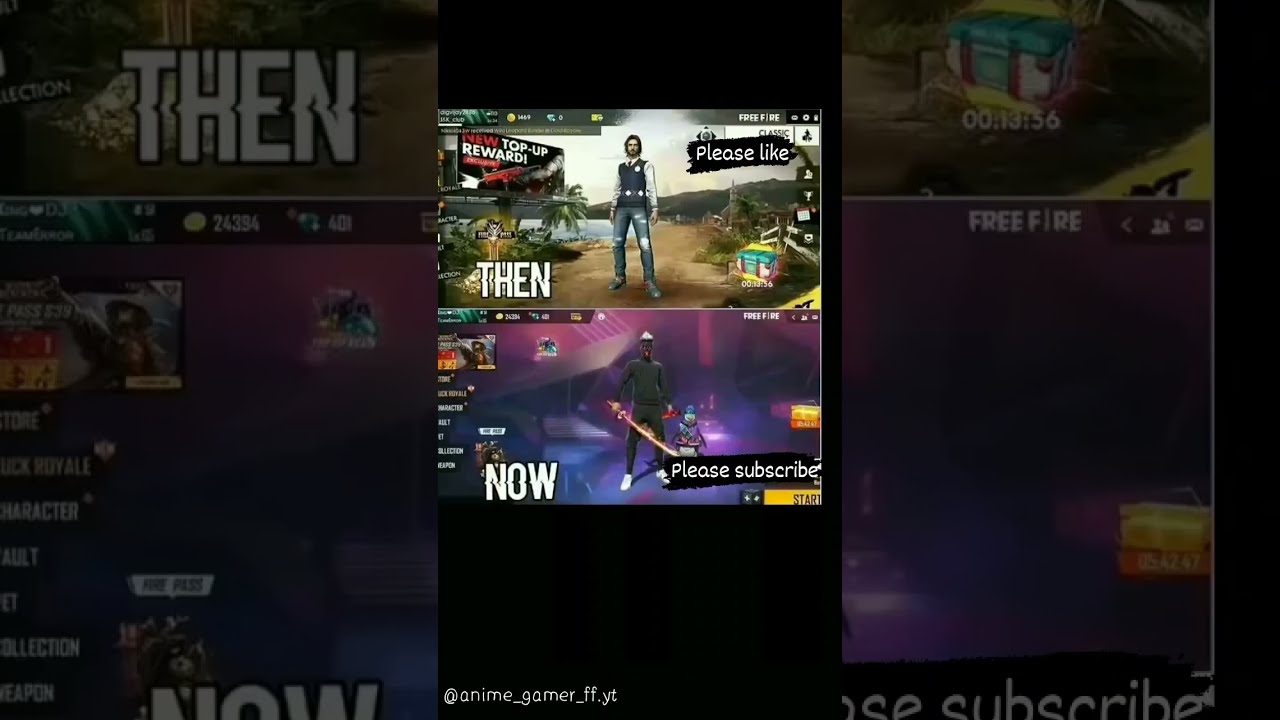This is a vertical cell phone-style image showcasing a comparison screenshot from a video game, likely sourced from a streaming platform. The image is bordered on the top and bottom by black rectangles, with the bottom one being wider. In the bottom left-hand corner of the wider black rectangle, there is a small piece of text that reads "@anime_gamer_ff.yt" in white font. The main image is divided into two sections: the top labeled "then" and the bottom labeled "now," suggesting a comparison between an older version and an updated version of the game.

In the "then" section at the top, the image depicts a video game character standing on a dirt road in a jungle environment with a palm tree visible on the left side. The text "please like" appears on the right side. The character is dressed in black armor with a white shirt and blue jeans, and another text "new top up reward" is visible in the top left corner.

In the "now" section at the bottom, the image shows the same game character now standing in a multicolored rave-type room, suggesting a more vibrant and modern game upgrade. The character is now dressed in sweatpants and a sweater, holding a sword. The text "please subscribe" appears on the right side of this image.

Overall, this detailed comparison highlights the visual and environmental upgrades in the video game over time. The background consists of a zoomed-in and faded version of the same main image, creating a cohesive visual effect.